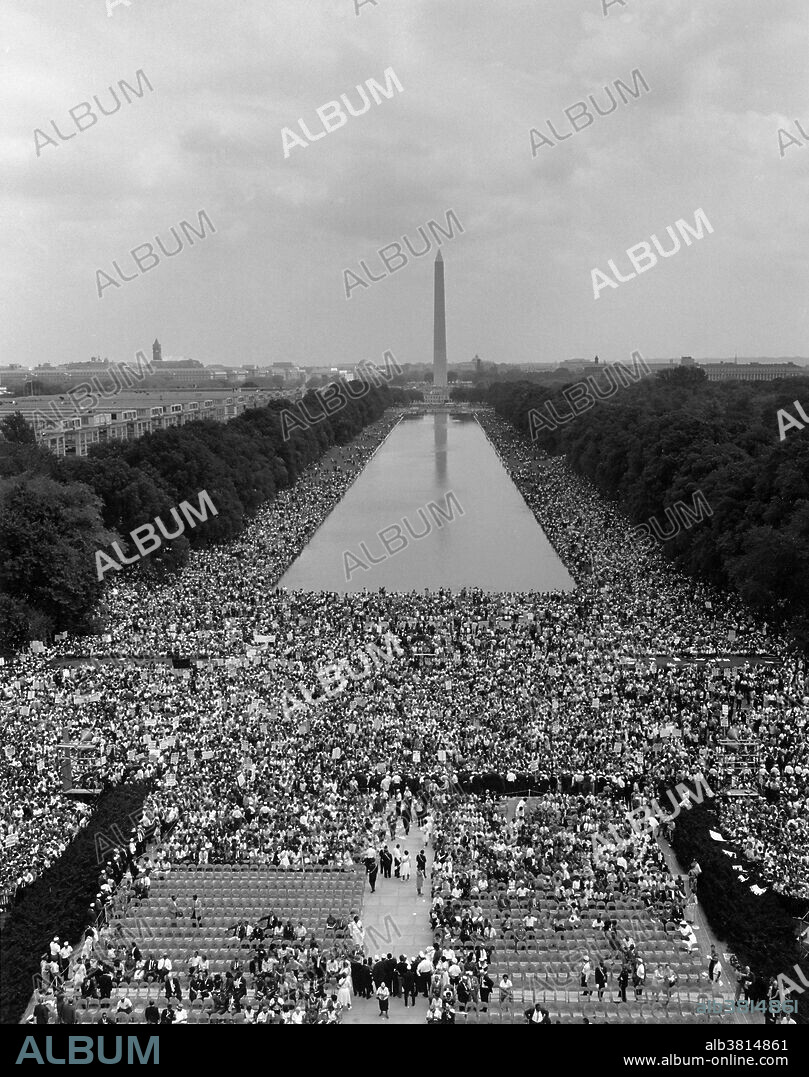The black-and-white photo showcases the iconic Washington Monument in Washington, D.C., prominently standing in the horizon with its reflective rectangular pond stretching in front of it. The scene captures a massive crowd of people, gathered densely around the water and extending far into the distance. In the foreground, a set of stairs, presumably for VIPs, appears largely emptied, suggesting the event has likely concluded. The perspective of the image seems elevated, offering a bird’s eye view of the bustling activity below. Surrounding the pond on either side are rows of trees, framing the lively scene. In the background, the tops of surrounding buildings and potentially historical row houses are faintly visible, adding depth to the urban landscape. Overlaying the entire image are numerous repetitions of the word "ALBUM" diagonally, with the website www.album-online.com clearly visible in the bottom corners.